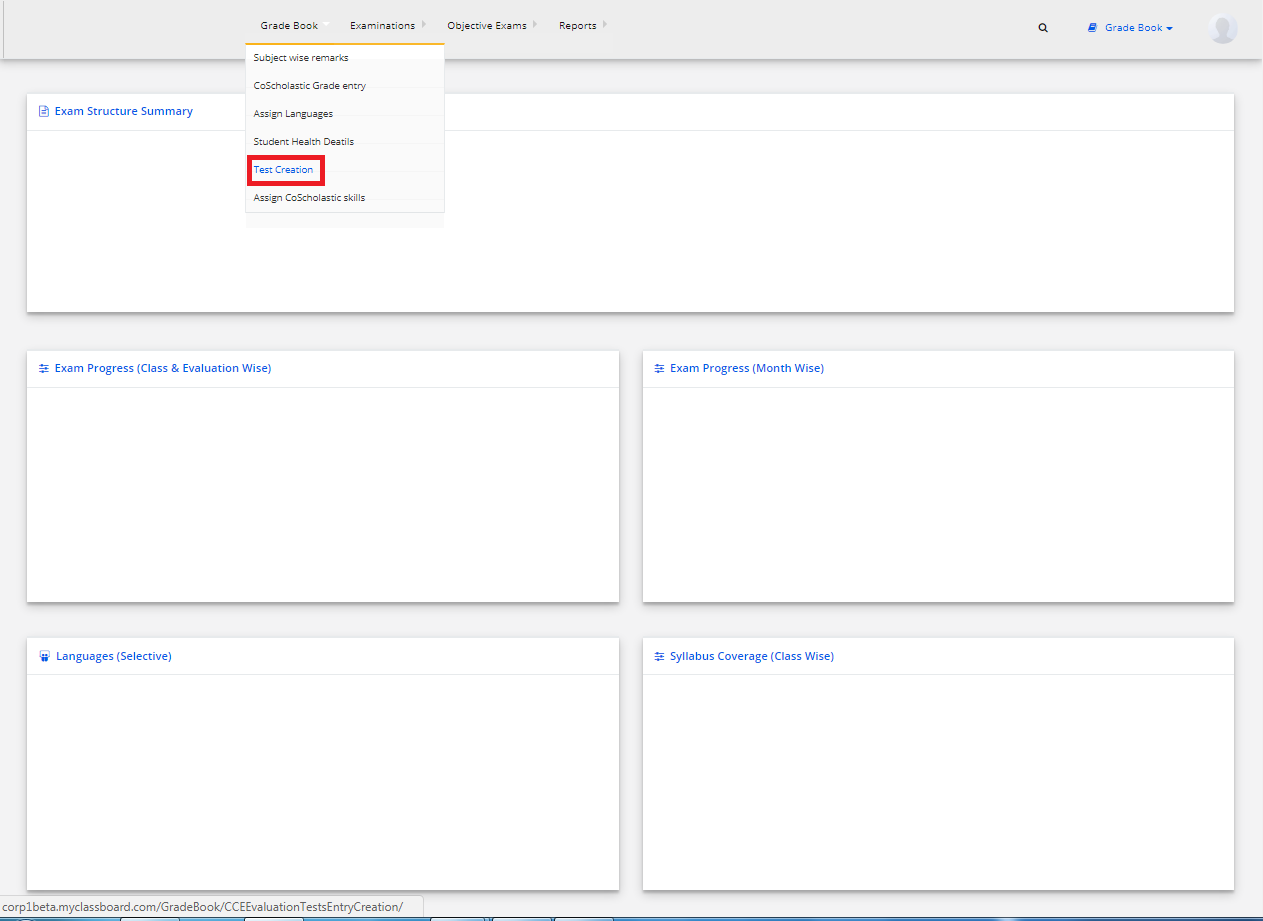The image depicts a predominantly white digital interface screen, designed likely for educational or administrative purposes. At the very top, there is a thin black header with very small text mentioning tabs such as "Gradebook," "Examinations," "Objective Exams," and "Reports." Below the "Gradebook" and "Examinations" tabs, there is a difficult-to-read drop-down menu. Although the first option is illegible, the third option appears to be "Assign Languages." The second-to-last option in this menu is highlighted in blue with a bold red outline, though its text remains unreadable.

In the upper right corner of the interface, another drop-down menu, this time fully visible in blue, is labeled "Gradebook."

Below these elements, on the left side of the screen, there is a long, thin input box stretching horizontally from left to right. In the upper left corner of this box, the text reads "Exam Structure Summary." Beneath this long input box is a large horizontal rectangle, divided in half to create two smaller rectangles side by side.

In the left of these two smaller rectangles, the text reads "Exam Progress Class and Evaluation Wise" with a subheading "Languages Selective," both written in blue. The right rectangle displays "Exam Progress Month Wise" with a subheading "Syllabus Coverage Class Wise," also in blue.

Overall, the interface seems to be a complex, multi-functional digital tool focused on exam and grade management, though its legibility is hampered by the small font size and color contrasts.